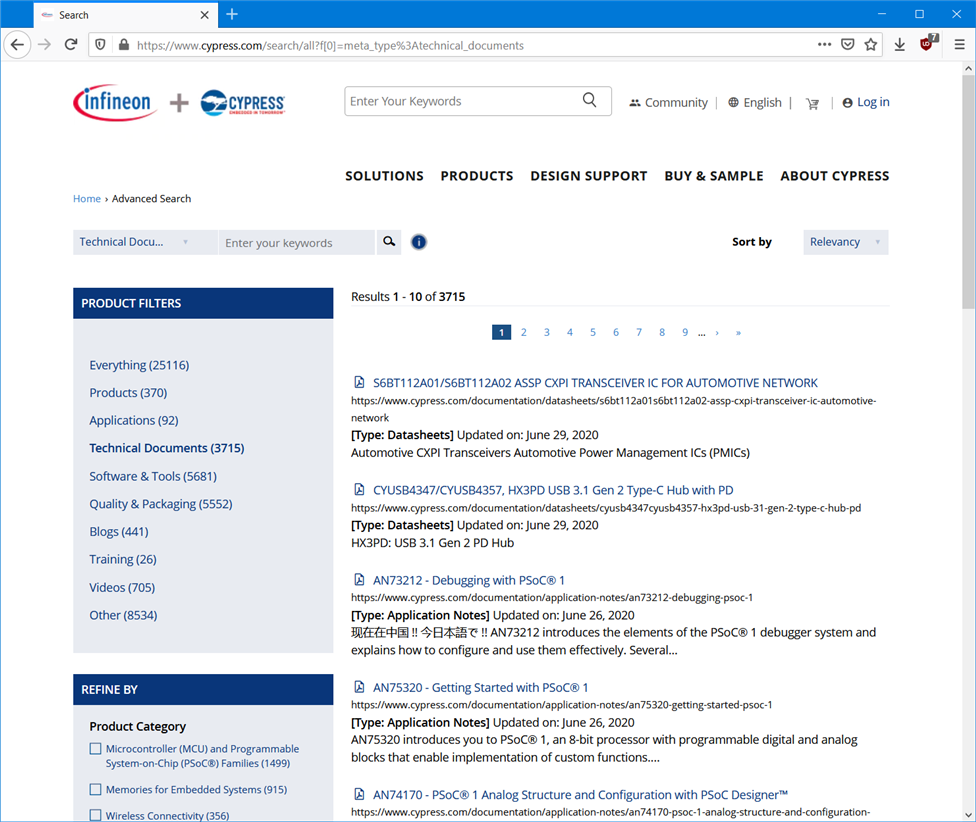This screenshot captures the main interface of the Infineon and Cypress website, cypress.com. The top banner prominently displays the Infineon + Cypress branding. Below the banner, a search bar is provided for keyword entry, coupled with navigation links for 'Community,' 'English,' 'Log In,' and several drop-down menus and clickable buttons labeled 'Solutions,' 'Products,' 'Design Support,' 'Buy & Sample,' and 'About Cypress.'

On the left sidebar, there are product filters and a section titled "Refine By" for narrowing down search results. The central part of the screen showcases the search results, indicating that it's displaying items 1 to 10 out of a total of 3,715 entries. The visible entries are listed numerically as 1 through 5, and the remainder can be accessed by scrolling vertically. To the right, a scrollbar is visible, suggesting more content below the fold. Additionally, pagination controls are located at the top of the search results, with the current page set to '1'. Subsequent pages can be accessed by clicking on the numbered links, which range from 1 to 9, with the option to continue beyond these initial pages.